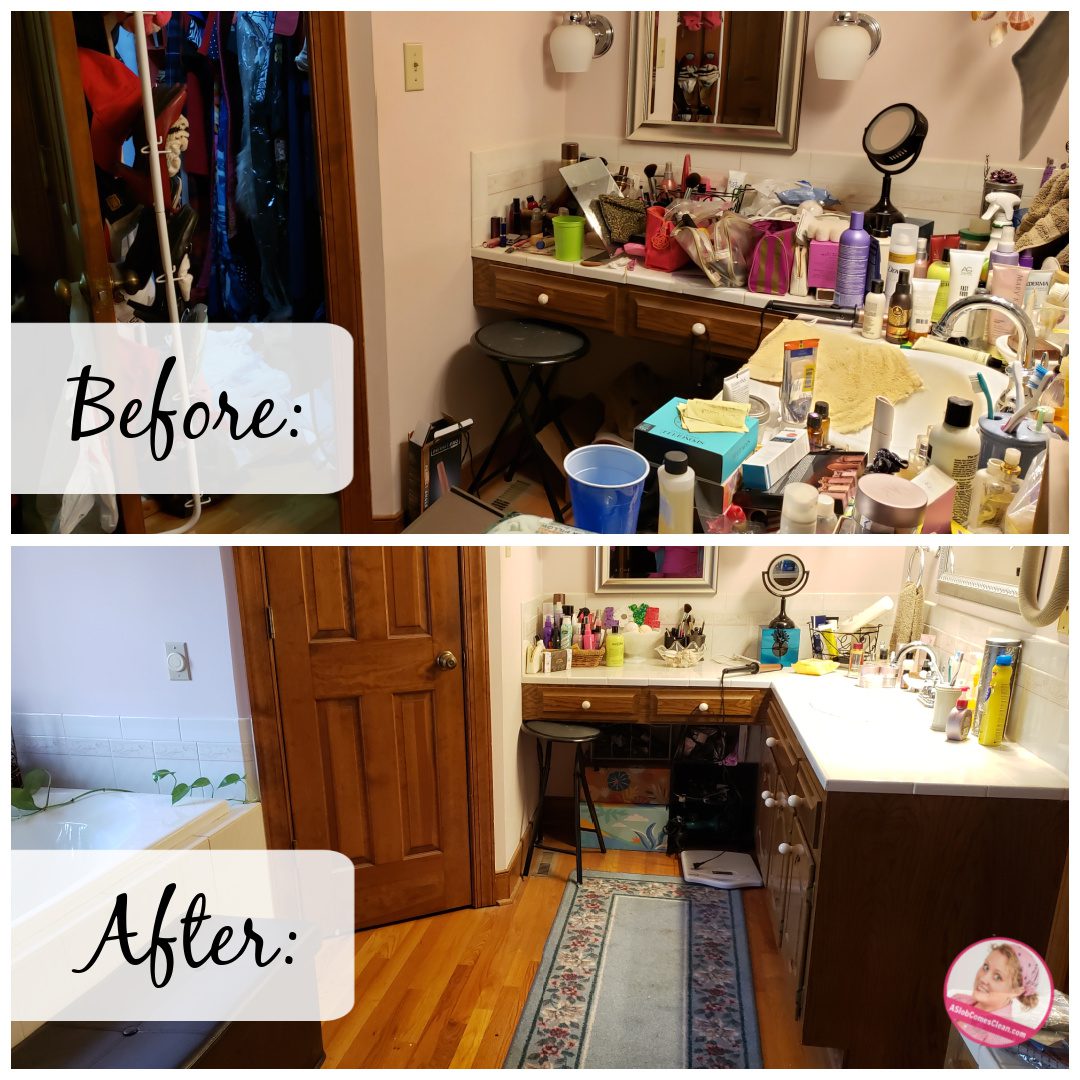This image appears to be an Instagram post showcasing a dramatic before-and-after transformation of a bathroom. The photo is horizontally divided, with the top half depicting the "before" state, and the bottom half illustrating the "after" state. In the cluttered "before" section, an L-shaped countertop on the right is cluttered with various bottles, cups, cosmetic brushes, and a toothbrush holder. Colors range from pink and purple to green. The scene also includes a black framed mirror, a shower curtain with shades of blue, black, and red, and a blue trash can. The wall is a pinkish color, and text that reads "before" is visible in black letters on a white triangle in the left-hand corner. 

The "after" section shows a dramatic improvement. The shower curtain is gone, revealing a clean white wall and tiles, and possibly a bathtub. The countertops are now organized and neat, with white tops and brown cabinetry that features white knobs. Items are neatly arranged along the wall. A pale blue oriental rug with floral edges is now in front of the cabinetry, and a white scale is placed on the floor. The text "after" is situated in the lower-left corner in black letters. A small circle at the bottom right corner encloses the image of a woman with her hair tied back, possibly the person who did the cleaning, making this a polished social media post.